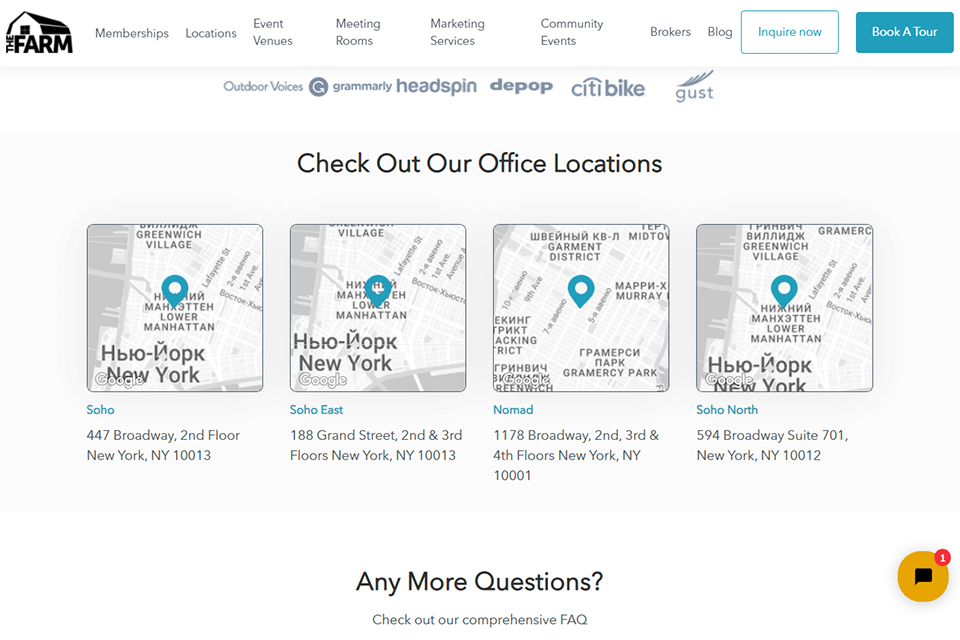The top section of the image features a white background with the text "The Farm" in black, positioned on the left-hand side. Above this text is a simplistic, black-and-white depiction of a barn. Below, in black text, is a list of services including "Memberships, Locations, Event Venues, Meeting Rooms, Marketing Services, Community Events, Broker's Block."

Beneath these, there are two prominent rectangles: the first has a white interior with a teal border and contains the text "Inquire Now" in teal; the second rectangle is teal with the text "Book a Tour" in white. The encompassing background of the image is light gray.

Further down, there is a list of company names in gray text: "Outdoor Voices, Grammarly, Headspin, D-Bob, City Bike, Gust." Below this list, in black text, it reads "Check out our office locations."

This section is followed by location information for various offices:
- **Soho**: 447 Broadway, Second Floor, New York, NY 10017 (in teal text)
- **Soho East**: 188 Grand Street, Second and Third Floors, New York, NY 10013 (in black text)
- **Nomad**: 1178 Broadway, Second, Third, and Fourth Floors, New York, NY 1001 (in teal text)
- **Soho North**: 584 Broadway, Suite 701, New York, NY 10012 (in black text)

At the bottom, a black text question reads "Any questions?" followed by "Check out our comprehensive FAQ" in black text. Adjacent to this, there is a black shield containing a red circle with a white number "1" inside it.